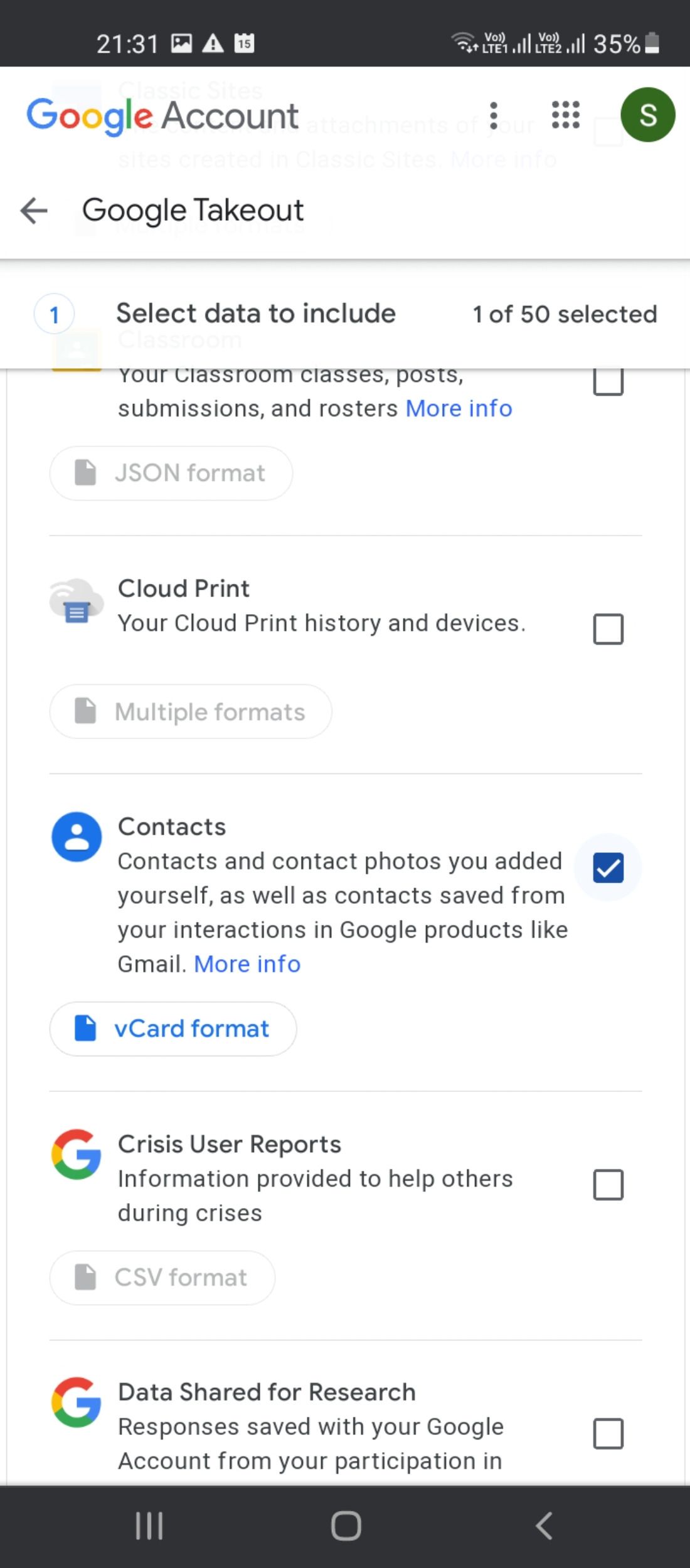This is a detailed screenshot from a smartphone. At the very top, there is a thin, black bar that spans the entire width of the screen. Within this bar, white text displays the time as 21:31, indicating it is 9:31 p.m. Positioned from left to right, there are several icons: a white photo, a white triangle with a black exclamation point, a white calendar, the Wi-Fi symbol, a phone signal strength icon, and a battery icon showing 35% charge.

Below this black bar, the Google logo appears in its signature multicolored format (blue, red, yellow, blue, green, and red), followed by the word "Account" in black text. On the right side, there are three vertical dots, indicating a menu, and next to these dots, a 3x3 grid of small dots forms a square. To the right of this, a green circle contains a white "S."

Underneath, a black arrow pointing left is followed by the text "Google Takeout" in black. Below this, a gray bar contains a gray circle with a blue number 1 on the left side, next to the text "Select Date to Include." To the right, it states "1 of 50 selected."

Further down, black text reads "Your Classroom Classes, Post, Submissions, and Rosters," with a "More Info" link in blue. Below this is a search bar, which features a gray icon resembling a folded piece of paper, with the label "JSON Format."

Underneath, an image of a gray cloud is associated with the text "Cloud Print" in black, followed by the description "Your Cloud Print History and Devices." There is another search bar below this, featuring a gray page icon and the label "Multiple Formats" in black. To the right of both options, there is an unchecked box.

Beneath these sections, a blue circle with a white person icon precedes the text "Contacts" in black. The description reads, "Contacts and Contact Photos You Added Yourself, as well as contacts saved from your interactions in Google products like Gmail." A "More Information" link appears in blue, with a checked box (blue with a white checkmark) to its right.

Another bar appears under this section, featuring the text "vCard Format" in blue, accompanied by a rainbow-colored "G" for the Google logo. Adjacent to this, in black text, it says "Crisis User Reports, Information Provided to Help Others During Crisis." There is a search bar below that labeled "CSV Format," with an unchecked box to its right.

Near the bottom, another Google "G" appears, followed by the text "Data Shared for Research" in black. The description states "responses saved from your Google account, from your participation in..." and then abruptly cuts off at the bottom where another inch-long black bar can be seen.